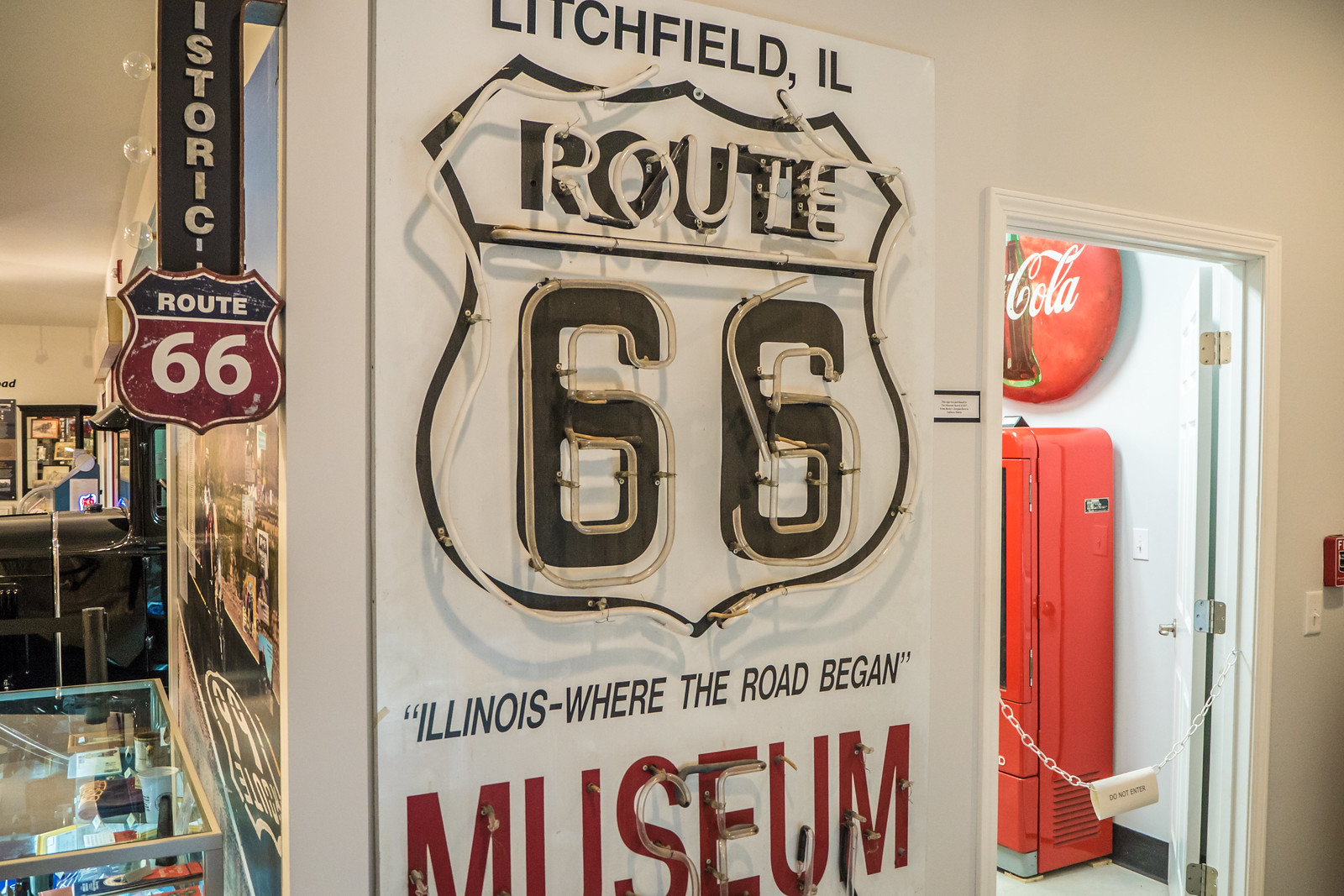This image captures an indoor scene at a museum dedicated to the historic Route 66, located in Litchfield, Illinois. The focal point of the image is a prominent black and white sign that reads "Litchfield, Illinois," with a neon inscription of "Route 66" beneath it, followed by "Illinois, Where the Road Began" and "Museum" in large red letters. To the left, there is a vintage Coca-Cola vending machine alongside a classic Coca-Cola sign mounted on a white wall. A doorway is partially obstructed by a chain guard and bears a "Do Not Enter" sign, suggesting restricted access. Inside this museum room, an old black car from the 1930s or 1940s can be seen, adding to the historical atmosphere. Various Route 66 signs, including one in the iconic shield shape, emphasize the thematic focus on this legendary highway.